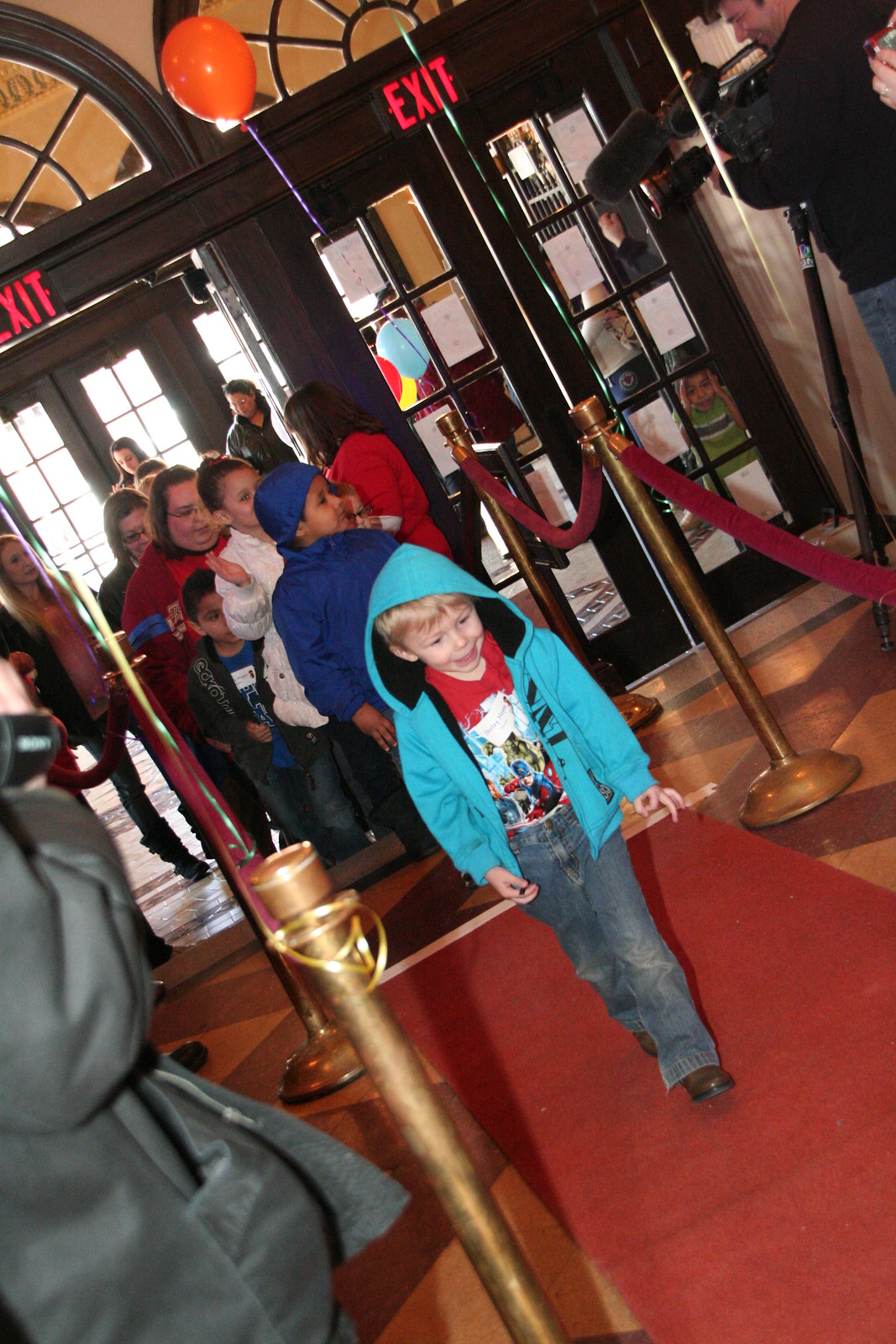The photograph captures an indoor scene at the entrance of a building, likely a movie theater or similar venue, with a red carpet flanked by velvet rope railings guiding visitors inside. Central to the image is a smiling young boy with blonde hair, wearing a light blue hooded jacket over a red Avengers t-shirt, blue jeans, and brown shoes, walking confidently down the red carpet. Surrounding him is a bustling scene of children and their parents, all making their way through a doorway marked by a red exit sign above. An orange balloon is tied to the beginning of the roped-off area, adding a touch of festivity. Onlookers, including a person taking photographs, are positioned outside the ropes, capturing the lively moment. Through a closed door, another child is visible, pressing his face to the glass, curiously peeking at the event unfolding inside. The setting is warmly lit with a rich color scheme of reds and browns, emphasizing the celebratory atmosphere as attendees arrive at the entrance.